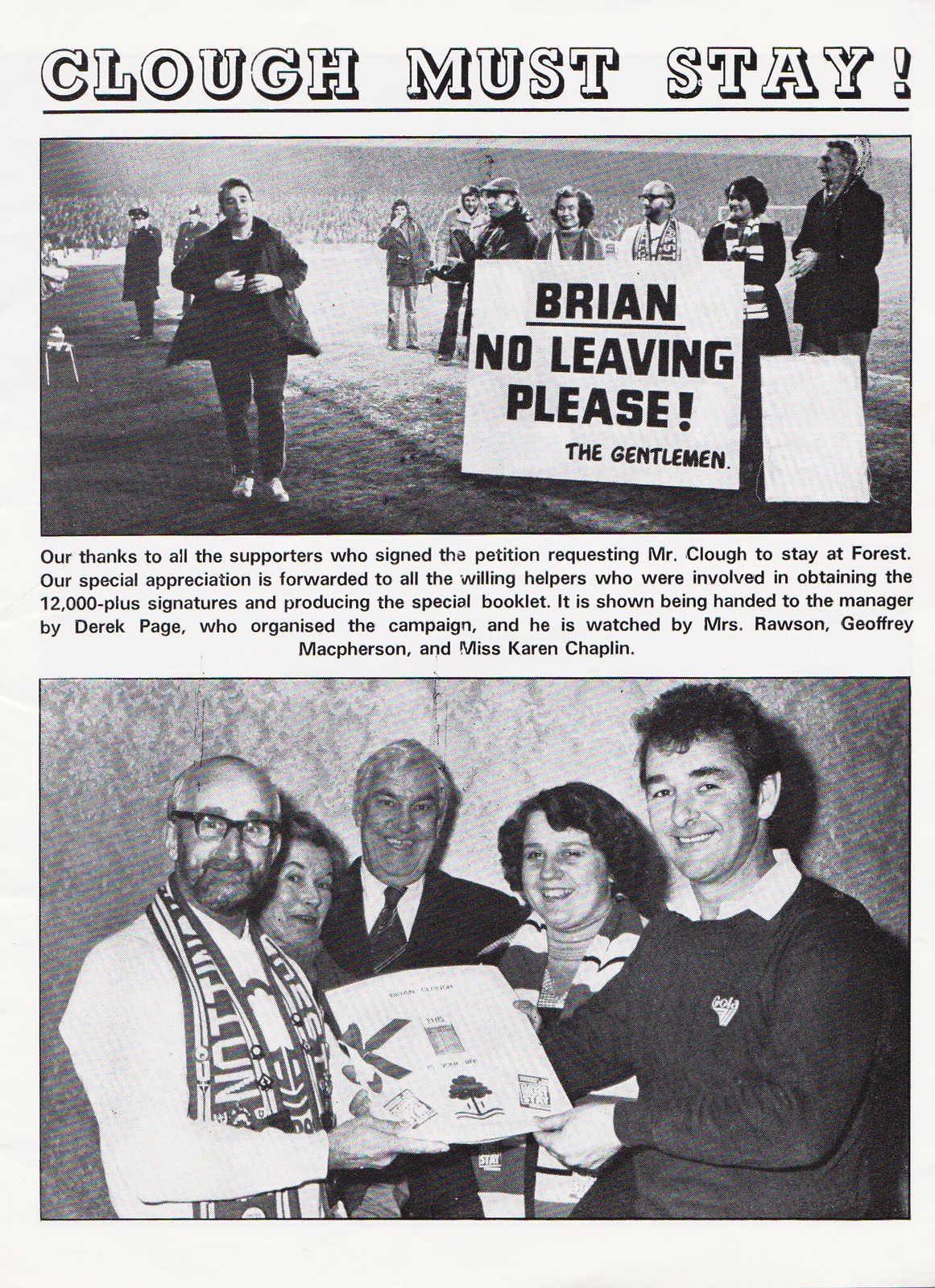The black-and-white magazine page is divided into two sections: the top section features a large photograph of several people standing on the left, behind them a big white sign reads "Brian, no leaving please." Above the photograph is the title "Klauf Must Stay!" in bold white letters on a black border. The bottom section contains another photograph showing five individuals, including Mr. Klauf, holding a square white object, which is a booklet. Between these photos is a body of text expressing gratitude to supporters. It reads: "Our thanks to all the supporters who signed the petition requesting Mr. Klauf to stay at Forest. Our special appreciation is forwarded to all the willing helpers who were involved in obtaining the 12,000-plus signatures and producing the special booklet. The booklet is shown being handed to the manager by Derek Page, who organized the campaign, and is watched by Mrs. Rawson, Jeffrey Macpherson, and Ms. Karen Chaplin."